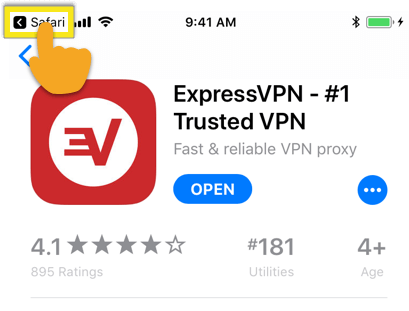The image depicts a screenshot of the ExpressVPN app listing on the iPhone App Store. A clipart icon of a hand is positioned over the screen, clicking the "Go to Safari" button. The status indicators at the top of the screen show strong signal strength, a connected Wi-Fi network, a time of 9:41 a.m., active Bluetooth connection, and a fully charged battery. 

The app icon is red and features a combined reverse "E" and "V" logo. The title reads "ExpressVPN – #1 Trusted VPN" and is followed by a descriptor in grayed-out text stating "Fast and reliable VPN proxy."

Additional elements on the screen include a circle with three dots for more options and a blue, pill-shaped "OPEN" button in white font. The app has a rating of 4.1 out of 5 based on 895 ratings. It is listed as number 181 in the Utilities category and is recommended for users aged 4 and up.